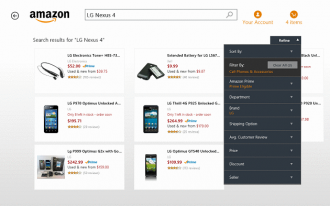The image is a screenshot of an Amazon search results page for the query "LG Nexus 4." At the top of the screen, the search bar displays the text "LG Nexus 4," with the Amazon logo and a backward arrow to the left of the search box. To the right, there is an option labeled "Your Account" followed by the text "search results for LG Nexus."

The visible portion of the page contains eight product images, although they are significantly blurred, making details difficult to discern. The first image appears to be an accessory, while the second and fifth images seem to depict a phone. The third image shows a phone along with accessories, and the fourth image appears to be a phone case. The sixth image is another phone.

The seventh and eighth images are partially obscured by a drop-down menu, which has been accessed by hovering over an option. This menu, rendered in dark blue and black tones, contains ten options, including "Sort by" and "Average Customer Review." However, the majority of the text within the menu is too blurry to read. Overall, approximately 80% of the image is blurred, obscuring finer details.